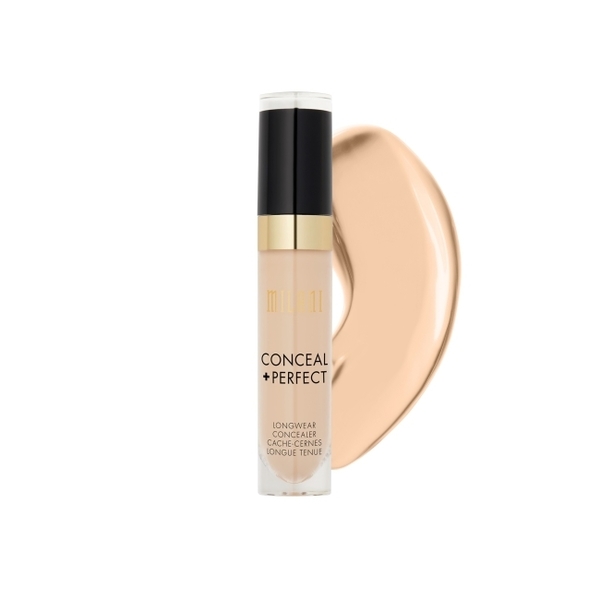The image showcases a single tube of concealer prominently centered against an all-white background, which gives it a minimalist, clean aesthetic suitable for a makeup advertisement. The concealer comes in a tall, clear container, revealing its beige, flesh-toned product inside. The tube is capped with a black lid accented by a gold band at its base. The bottle features text in black, stating "CONCEAL + PERFECT," followed by "LONGWEAR CONCEALER," "CACHE CERNES," and "LONGUE TENUE," indicating its extended wear and multilingual labeling.

To the right of the tube, there is a thick, curved smear of the beige concealer, giving a visual representation of its color and texture. The smeared product arcs gracefully from behind the black lid, moving downwards and narrowing as it extends behind the bottom part of the tube. This swatch appears to be applied with a brush, providing a realistic depiction of how the concealer looks when used. The overall presentation, with its clear product visibility, elegant labeling, and clean background, is indicative of high-quality, polished promotional imagery often found in magazines or online advertisements.